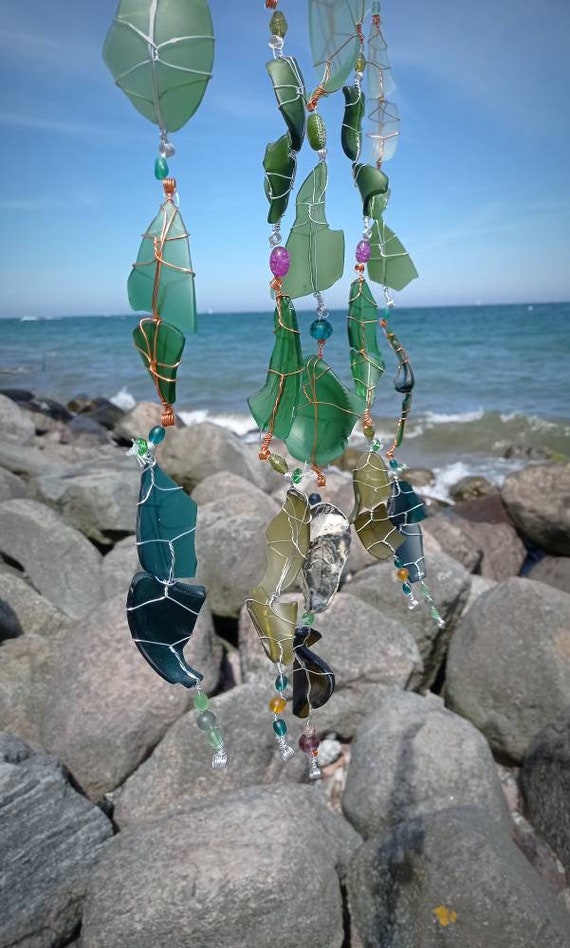In this image, the centerpiece is a wind chime crafted from recycled sea glass and adorned with colorful beads, all intricately connected by metal wiring. The chime, appearing as a delicate, luminous mobile sculpture, is suspended above a rugged, jetty-like formation of large, rounded and pointy stones on a serene beach. The ocean waves crash into these rocks, creating white breakers that add dynamism to the scene. Beyond the rocks, the vast expanse of water stretches out to meet a beautiful blue skyline dotted with wispy white clouds, capturing a tranquil, coastal atmosphere. The main focus remains the wind chime, set against this picturesque beach and ocean backdrop.